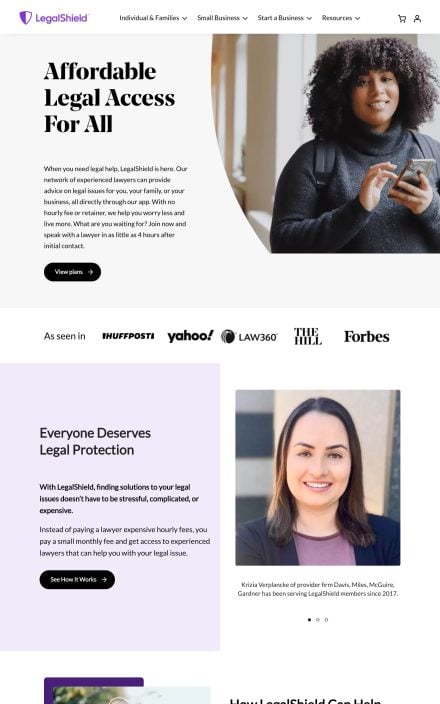The image displays a well-designed and modern webpage from LegalShield, featuring a prominent focus on providing affordable legal access to individuals and businesses. The LegalShield logo is distinctly positioned in the top left corner of the page. The top navigation bar includes links categorized for Individuals and Families, Small Business, Start a Business, and Resources. Additionally, there are icons for a shopping cart and user account located in the top right corner.

On the left side of the page, bold text reading "Affordable Legal Access for All" is prominently featured. Below this heading, a paragraph emphasizes the ease of access to legal advice and assistance provided by LegalShield. A conspicuous "View Plans" button is situated just below the paragraph.

To the right, an image showcases a smiling woman dressed in a dark sweater, holding a cell phone in her hand, with a backpack slung over her shoulder, conveying approachability and practical usability of the services.

Further down the page, the phrase "As Seen In" precedes notable publication logos including Yahoo!, Law360, The Hill, Forbes, and Huffington Post, reinforcing the company’s credibility. Accompanying text states "Everyone Deserves Legal Protection," with an explanatory paragraph below detailing how LegalShield offers simple and affordable legal solutions. A "See How It Works" button is positioned immediately below this descriptive paragraph.

Towards the bottom right, a photograph of Krista Wenzel, a LegalShield provider since 2017, is displayed alongside a brief description of her service, enhancing the personal touch and reliability of the platform.

While the current view limits visibility of additional subsections, the overall webpage design prioritizes trustworthiness, simplicity, and accessibility, effectively communicating the value of LegalShield’s legal services in a clear and concise manner. Further scrolling is likely to reveal more detailed information about LegalShield’s offerings and user experiences.